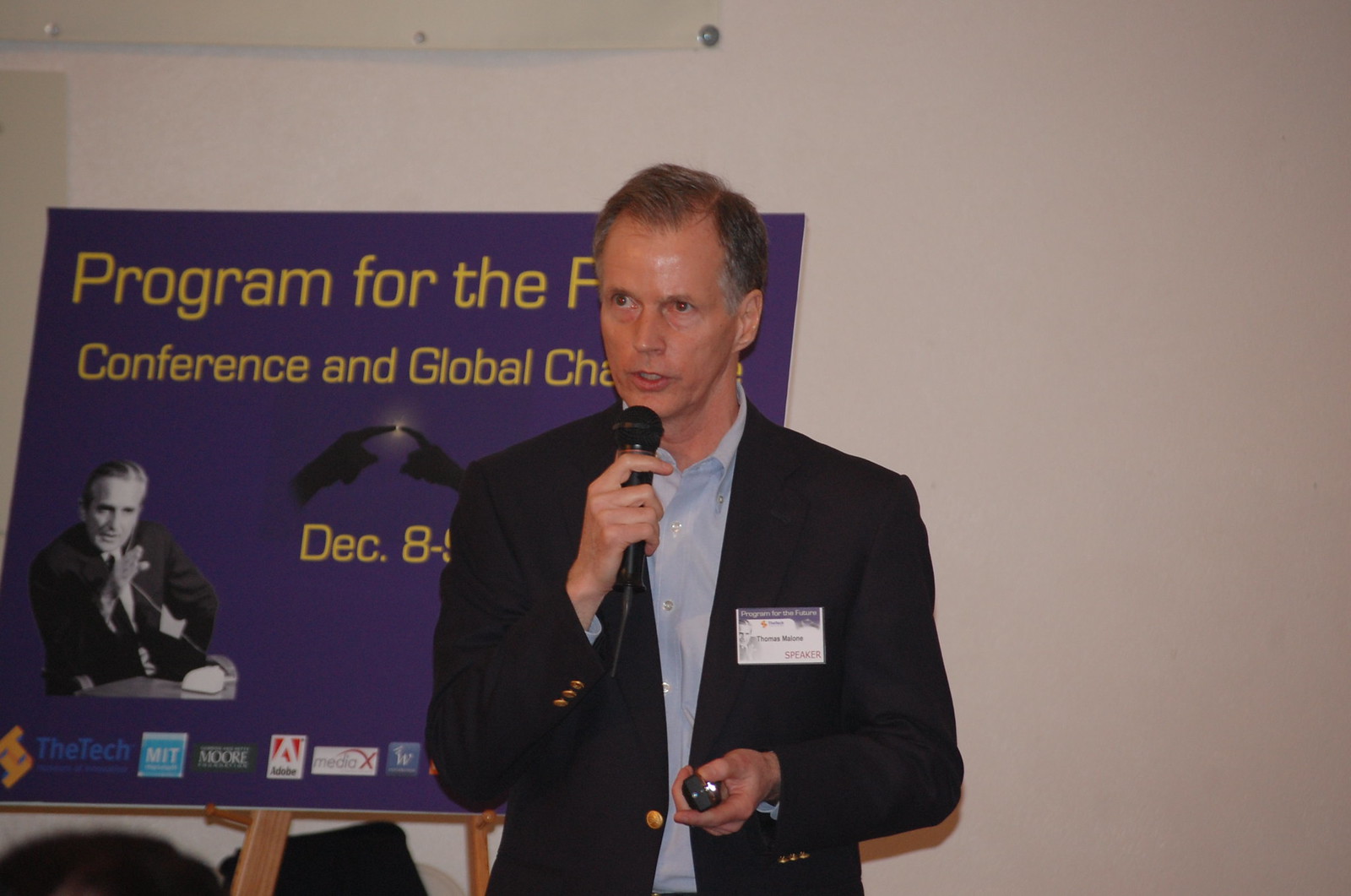In the center of the photograph, a man is speaking at a conference, holding a black microphone in his right hand. He is attired in a dark suit, a light blue shirt, and has a name tag on his left chest. Appearing to be in his late 50s, with graying hair, he is captured mid-sentence, his mouth open. He appears to be holding a remote to change slides in his other hand. Standing in front of a white wall, there is a purple poster on the left side of the image, displayed on a wooden easel. The top part of the poster reads "Program for the…" though it is partially obscured by the man's head, with visible text beneath saying “Conference and Global Change” and the dates “December 8-9.” The right side of the wall remains bare, while the man's stance and gaze suggest he is looking slightly to the left.